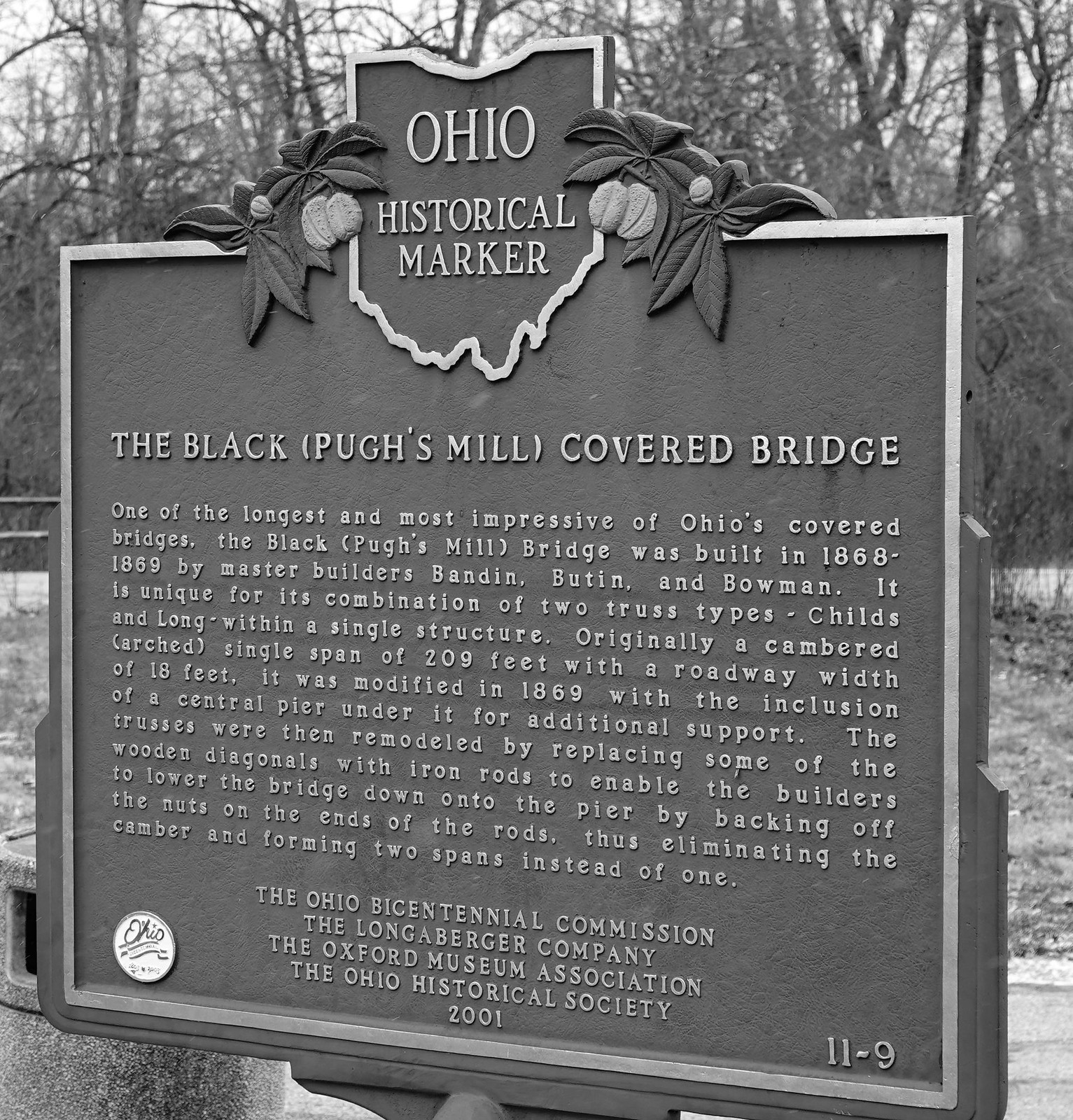This black-and-white photo captures a historical marker at an outdoor venue during winter, evidenced by the barren trees in the background. The metal plaque is prominently topped with the outline of the state of Ohio, flanked by Buckeye emblems. It reads "Ohio Historical Marker" and details the Black Pews Mill Covered Bridge. Described as one of Ohio's longest and most impressive covered bridges, it was constructed between 1868 and 1869 by master builders Bandon, Boutin, and Bowman. The bridge is noted for its unique combination of two truss types—Child's and Long—within a single structure. Originally a cambered single span of 209 feet with a roadway width of 18 feet, it was modified in 1869 with the addition of a central pier for extra support. This modification involved replacing some wooden diagonals with iron rods, allowing the bridge to be lowered onto the pier by adjusting the nuts, effectively eliminating the camber and creating two spans instead of one. The marker was erected in 2001 by the Ohio Bicentennial Commission, the Longaberger Company, the Oxford Museum Association, and the Ohio Historical Society. An emblem is situated on the bottom left of the marker, while "11-9" is inscribed on the bottom right.